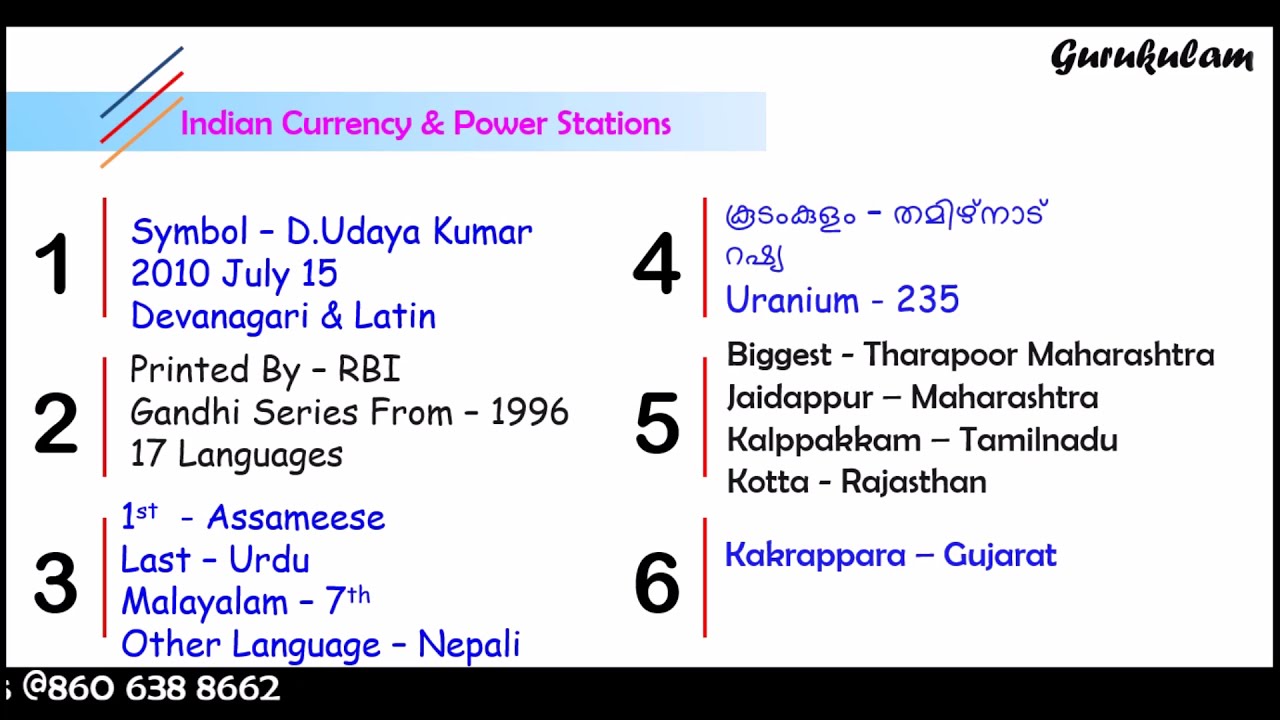The image displays an informational card with a header reading "Indian Currency and Power Stations." The title is written in pink font on a blue rectangular banner that features three diagonal lines in blue, red, and yellow. At the top of the image, there is the word "GURUKULAM," written in capital letters. The card has a numbered list from 1 to 6, each entry providing specific details:

1. "Symbol, D. Udaya Kumar, 2010, July 15, Devanagari in Latin."
2. "Printed by RBI, Gandhi Series from 1996, 17 Languages."
3. "First, Assamese; Last, Urdu; Malayalam, 7th; Other Language, Nepali."
4. "Uranium 235."
5. "Biggest: Tharapur, Maharashtra; Jaidapur, Maharashtra; Kalpakkam, Tamil Nadu; Kota, Rajasthan."
6. "Kakrapara, Gujarat."

The text on the card is in purple, blue, and black colors, presenting the information clearly and systematically. At the bottom, a contact number "860-638-8662" is also included.